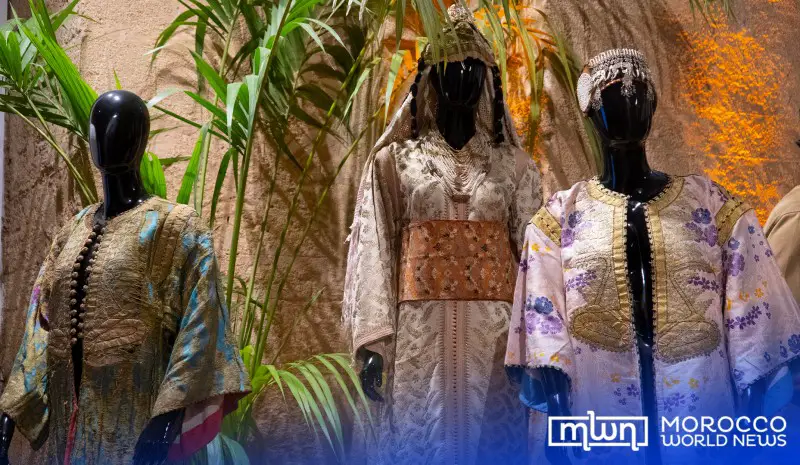In this photograph, three black mannequins stand against a white textured wall with lush green palm trees in the background. Each mannequin displays traditional, floral-themed tribal outfits. A text overlay at the bottom right corner reads "MWN Morocco World News" in a stylish blue and white font with a logo enclosed in a rectangular border.

The leftmost mannequin is adorned in a vest-like garment that ties in the front, featuring golden blue and floral designs with long, flowing sleeves. The middle mannequin sports a tan hat and a predominantly white outfit, accented with a darker tan and white patterned belt. Lastly, the rightmost mannequin is clad in a mostly white gown, detailed with goldish-blue floral patterns and a white cap, and it exhibits a yellow smudge that seems accidentally painted on.

The image captures the intricate, handcrafted look of these niche garments, emphasizing the artisanal effort and detailed designs, suggesting they may come from a smaller, dedicated business.